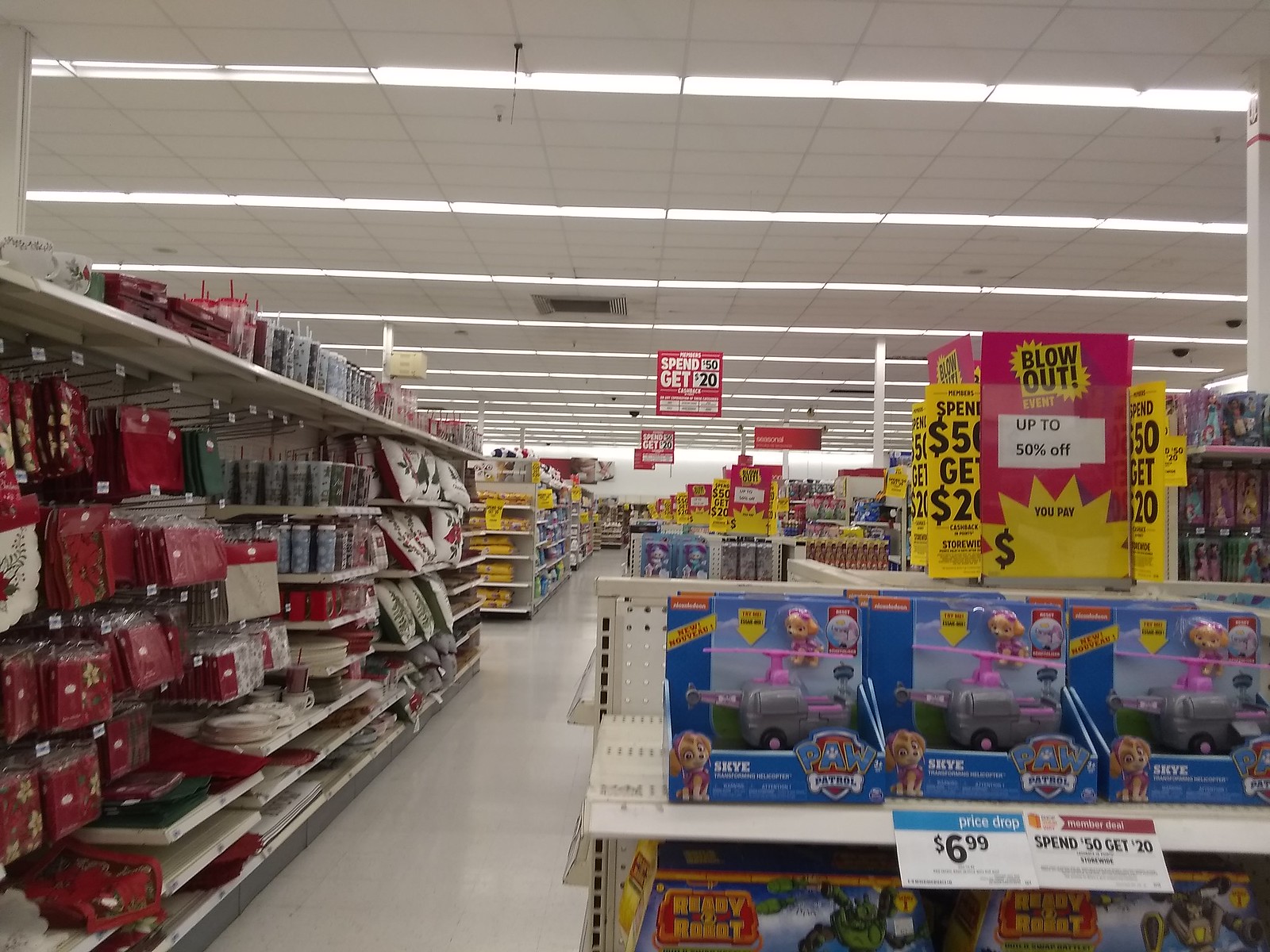In the image, we are immersed in a bustling grocery store setting that extends deeply into the background. At the forefront, there is a rack prominently displaying various toys. This rack features a bright blue tag indicating a "Price Drop," marking the toys down to $6.99. Beside this, there is a black text notice stating, "Spend $50, get $20." 

Below the display rack, additional toys are scattered. To the left, a series of red napkins catches the eye, contributing to what appears to be a Christmas-themed aisle, dominated by vibrant red, white, and green colors. Adding to the festive theme, signs overhead declare "Blowout Up to 50% Off" in striking yellow and red. Additionally, a large red sign is suspended from the ceiling, highlighting promotional offers. 

The scene continues with an array of aisles receding into the distance, teeming with various products. The ceiling above is composed of gray square tiles, interspersed with horizontal lines of white lights, efficiently illuminating the entire store.